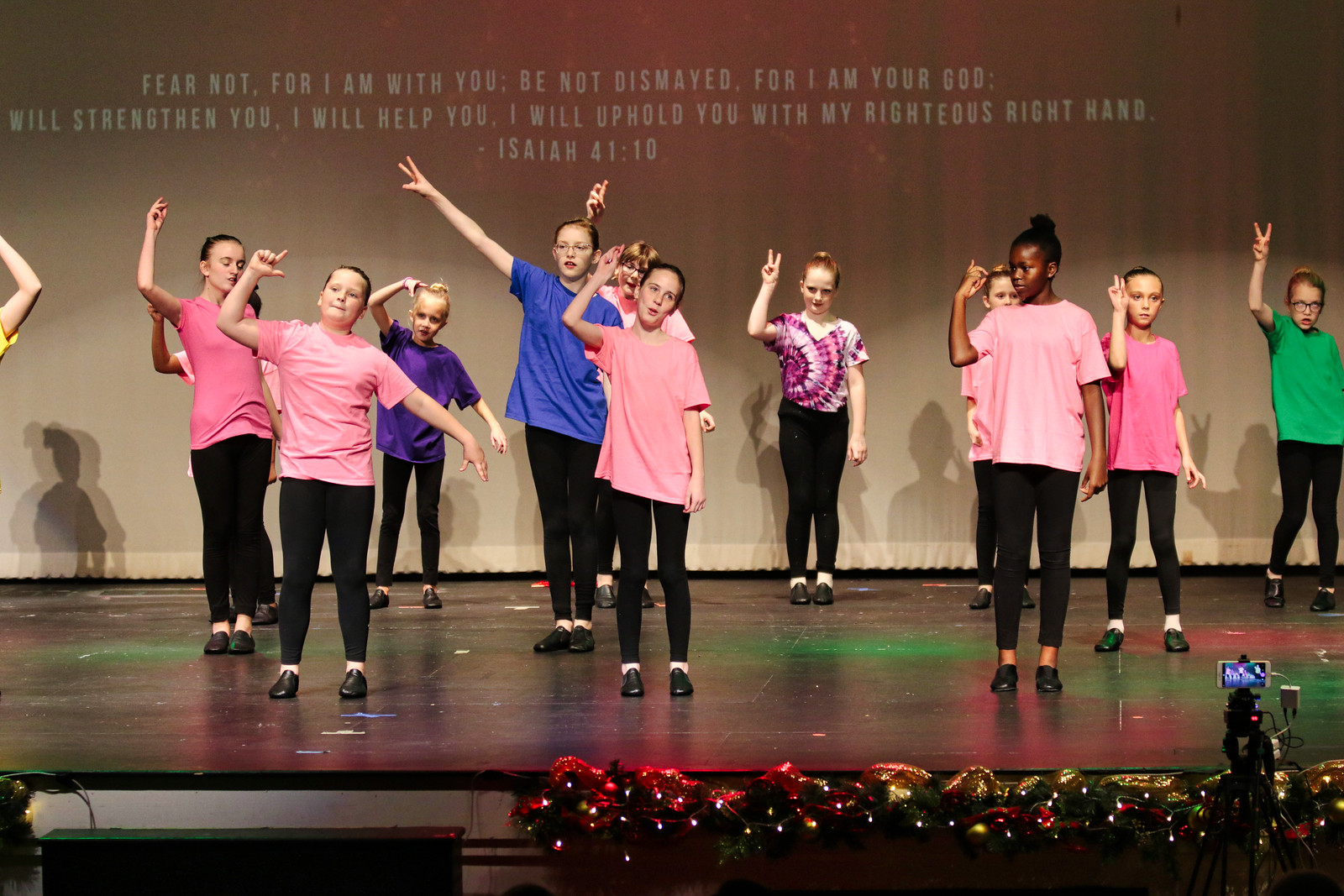The image captures a vibrant performance by young girls and boys, likely aged 10 to 13, on a wooden stage. The participants are uniformly dressed in black leggings and varied, colorful t-shirts—primarily shades of pink, but also including blue, green, purple, and a tie-dye of purple and white. Each performer is holding their right hand up in the air, bent at the elbow, mimicking the pose described in the biblical passage prominently displayed behind them. The backdrop features a brown background with white lettering quoting Isaiah 41:10: "Fear not, for I am with you; be not dismayed, for I am your God. I will strengthen you, I will help you, I will uphold you with my righteous right hand." Below the stage, festival lights illuminate the area, and a cell phone on a stand is actively recording the performance, capturing the youthful energy and the inspirational message of the event.